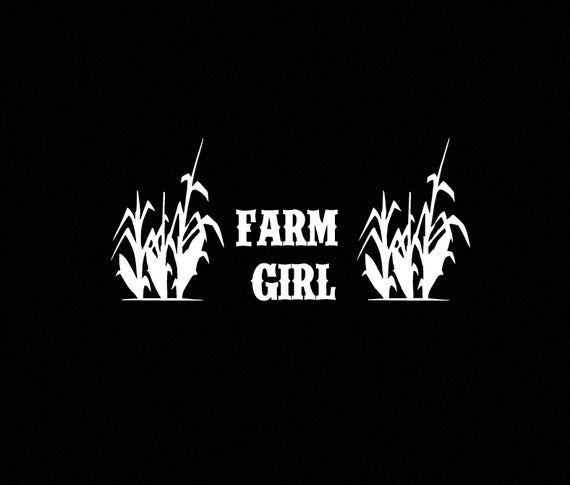The image features a black rectangular background in a landscape orientation. Centrally positioned, the bold and capitalized words "FARM GIRL" are stacked one above the other in a Western-style font, with their right edges aligned. Flanking the text are identical white silhouettes depicting three corn stalks in a row on each side, emerging from a line that indicates the ground. Notably, the middle stalk on the right side is taller than the others. The overall design is a black-and-white illustration that combines line art with typography, giving it a distinct and striking appearance.